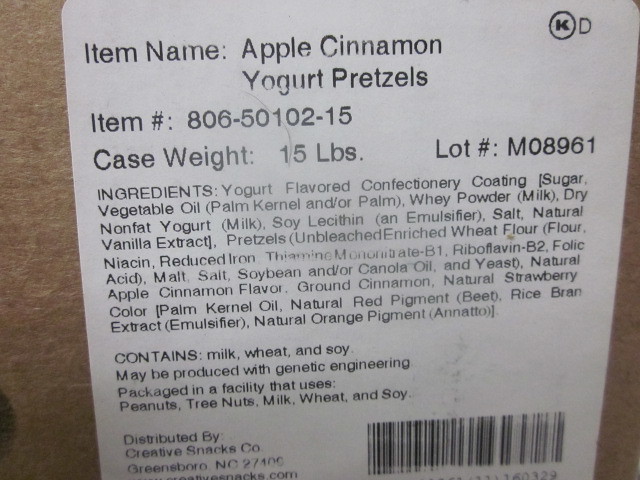The image showcases a close-up of a white label with black text for a product named Apple Cinnamon Yogurt Pretzels. The beige background contrasts with the label, which dominates the image. At the top left, the label reads "Item Name: Apple Cinnamon Yogurt Pretzels." Beneath this, it lists the item number as 806-50102-15. The case weight is stated as 15 lbs, and the lot number is M08961. The middle of the label features detailed ingredients, including yogurt-flavored confectionery, sugar, vegetable oils (palm kernel and/or palm), wheat powder, nonfat dry milk, soy lecithin, emulsifier, salt, and natural vanilla extract. The allergen information follows, highlighting that the product contains milk, wheat, and soy, and is packaged in a facility that uses peanuts, tree nuts, milk, wheat, and soy. Additionally, there is a note about potential genetic engineering. The bottom left corner holds distribution details, while the right lower corner includes a partially visible barcode.